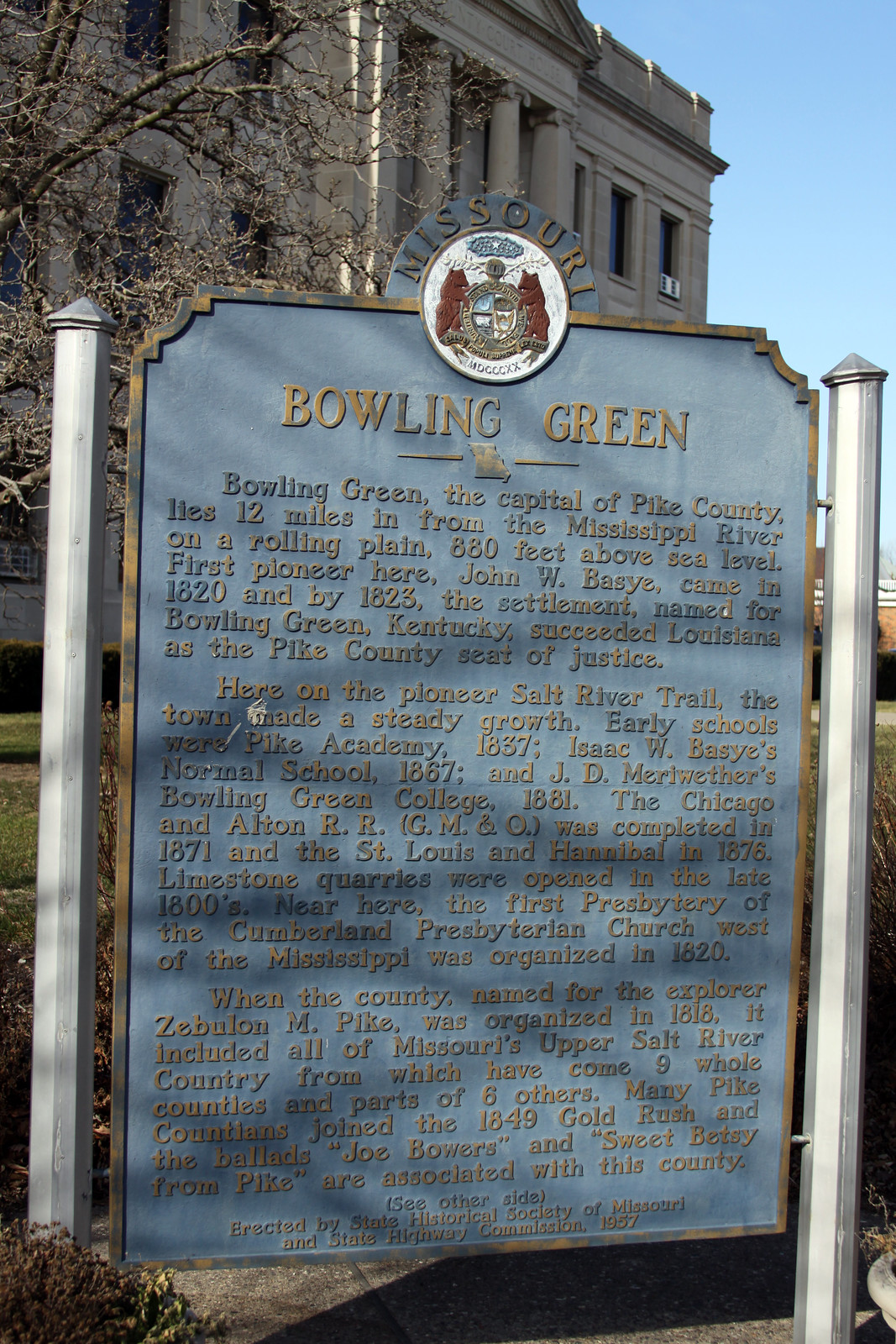This photograph, taken outdoors during the daytime, features a historical marker for the city of Bowling Green in the state of Missouri. The marker is situated on a metal sign supported by two thin metal posts with caps. The sign is placed against the backdrop of a tall white stone building with large columns, which occupies the top-left portion of the image. The background features a clear blue sky in the upper right-hand corner.

The historical marker, designed with an elegant curved top, has a blue background with raised gold or yellow print. At the top center of the sign is a white circular emblem bordered in gold, featuring the state seal of Missouri adorned with two bears and the word "Missouri" arching above it. Below the emblem, in prominent lettering, it declares "Bowling Green."

The text of the marker reads: 

"Bowling Green, the capital of Pike County, lies 12 miles in from the Mississippi River on a rolling plain, 880 feet above sea level. The first pioneer here, John W. Basye, arrived in 1820, and by 1823 the settlement, named for Bowling Green, Kentucky, succeeded Louisiana as the Pike County seat of justice. Here on the pioneer Salt River Trail, the town made steady growth. Early schools included Pike Academy (1837), Isaac W. Basye's Normal School (1867), and J.D. Meriwether's Bowling Green College (1881). The Chicago and Alton Railroad (G.M. and O.) was completed in 1871, followed by the St. Louis and Hannibal Railroad in 1876. Limestone quarries were opened in the late 1800s. Near this site, in 1820, the first presbytery of the Cumberland Presbyterian Church west of the Mississippi was organized. Pike County, named for explorer Zebulon M. Pike when organized in 1818, originally included all of Missouri's Upper Salt River Country, eventually giving rise to nine whole counties and parts of six others. Many Pike Countians joined the 1849 Gold Rush, and the ballads 'Joe Bowers' and 'Sweet Betsy from Pike' are linked to this area. See Other Side. Erected by the State Historical Society of Missouri and the State Highway Commission, 1957."

This marker not only provides a window into the rich history and steady development of Bowling Green, Missouri, but also highlights significant figures, institutions, and the spirit of exploration and growth that characterized the region.